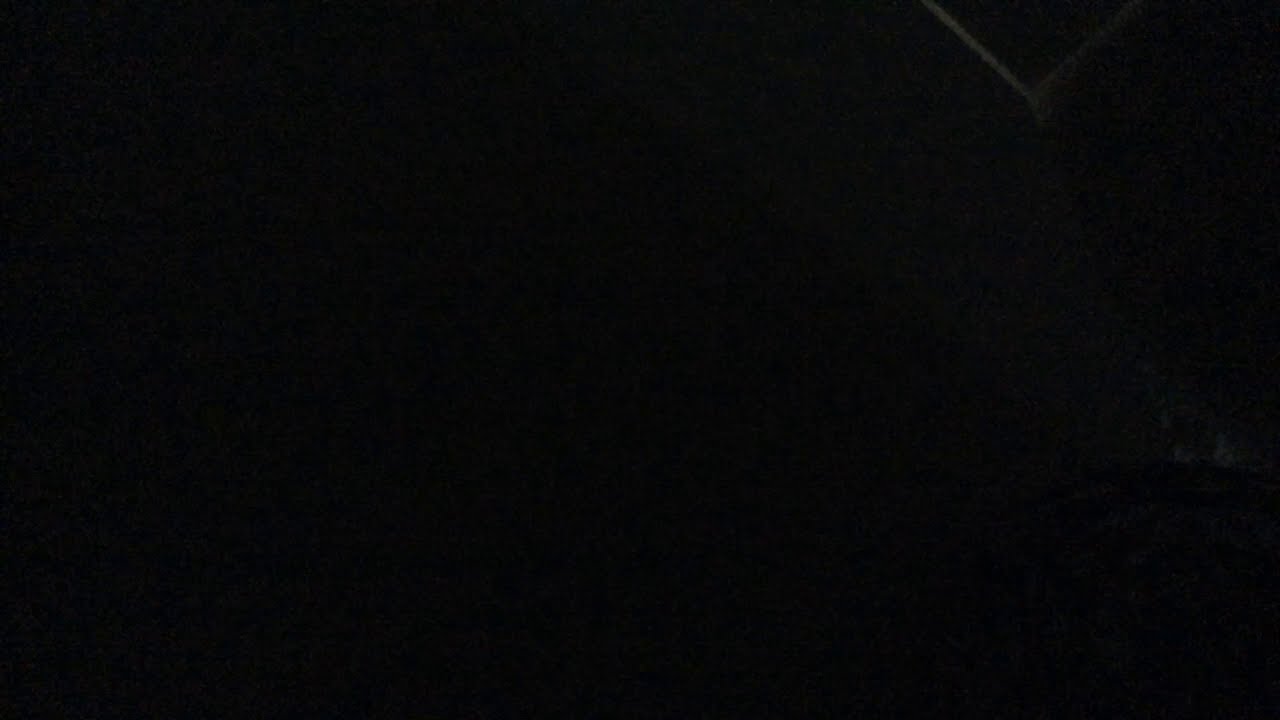The image is predominantly a pure black background, suggesting an error in the processing or exposure. In the upper right quadrant, roughly one quarter of the way over from the right edge, there's a faint gray streak extending downward at about a 40-degree angle. Additionally, along the right edge, slightly below the center, there is a faint gray smudge. There are no discernible objects or details due to the overall darkness of the image, with only these faint gray marks breaking the uniform black, possibly indicating a technical issue in capturing or developing the image.